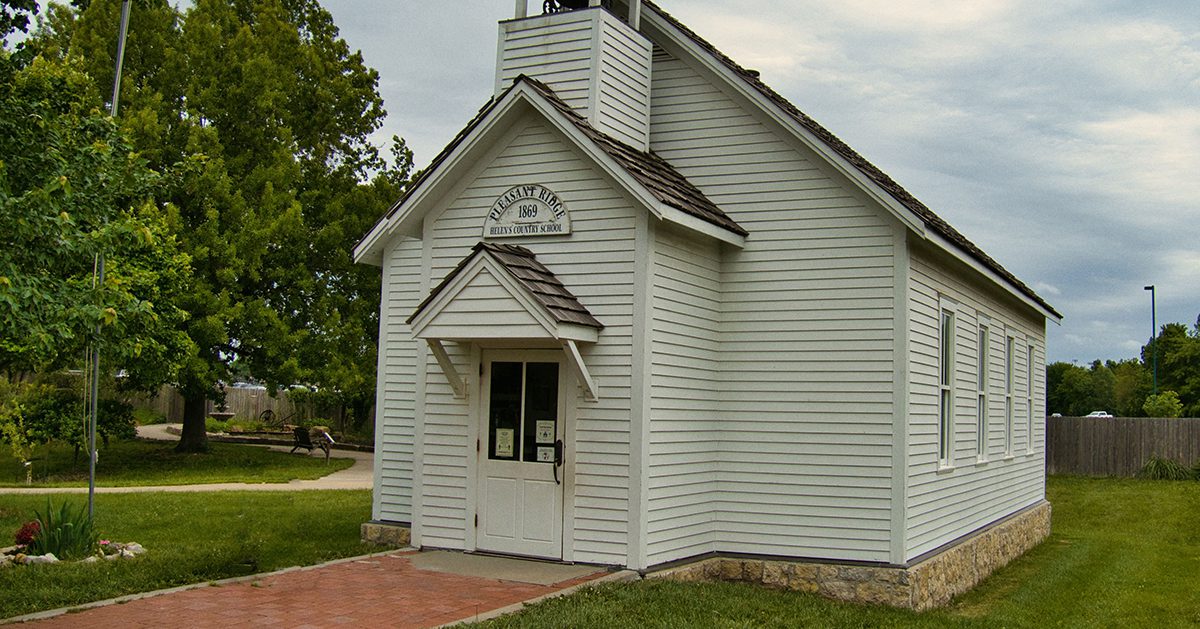This is a detailed color photograph, taken outdoors during the daytime, capturing a charming vintage one-room schoolhouse known as Pleasant Ridge Country School, established in 1869. The single-story building is well-preserved and modest, featuring white horizontal siding and a brown shingled, upside-down V-shaped roof. The entrance, set within a small pediment, is covered by an alcove to provide shelter from the elements. Above the entrance, an arched sign reads "Pleasant Ridge, 1869," although parts of the lower text, indicating it is a country school, are slightly illegible. 

The building has a series of four rectangular windows along one side. Extending from the lower left corner of the image, a red brick walkway leads visitors to the front door. There is greenery on both sides, with a well-kept garden and trees enhancing the picturesque scene. Behind the schoolhouse, the sky is a serene blue with scattered white clouds. The overall composition emphasizes the building's historical significance and its preserved state, likely maintained for museum purposes. The photograph's style falls under photographic representational realism, capturing the details and ambiance of this historical site.